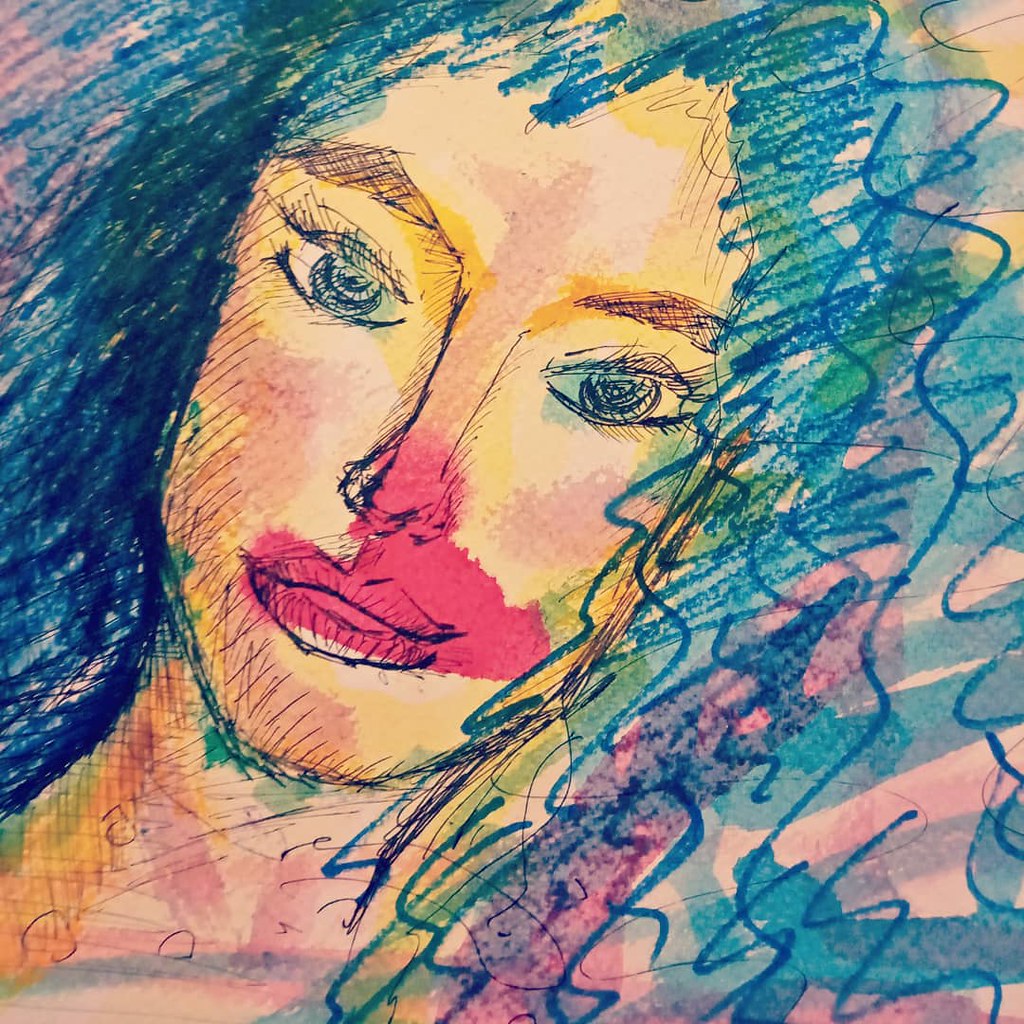This striking painting is an intriguing blend of watercolor and marker, capturing a portrait of an exotic and beautiful woman. Her long, black curly hair cascades down, accentuating her elongated, slender neck. Her large, almond-shaped eyes, adorned with long, dark eyelashes, convey a captivating intensity beneath her distinct eyebrows. Her full lips, dramatically smeared with lipstick that extends beyond their contours, spread across her face, touching above her top lip and over her nose, creating a surreal and arresting visual effect.

The artist has given her hair an imaginative twist; one side features bright blue, squiggly lines interwoven with pink, blue, and yellow watercolor, adding a vibrant, whimsical flair. In contrast, the left side of her hair is rendered with dense, straight lines in navy and light blue, providing a stark juxtaposition with its dense, thick texture. This combination of bold colors and contrasting styles contributes to the portrait's fascinating and otherworldly aesthetic.